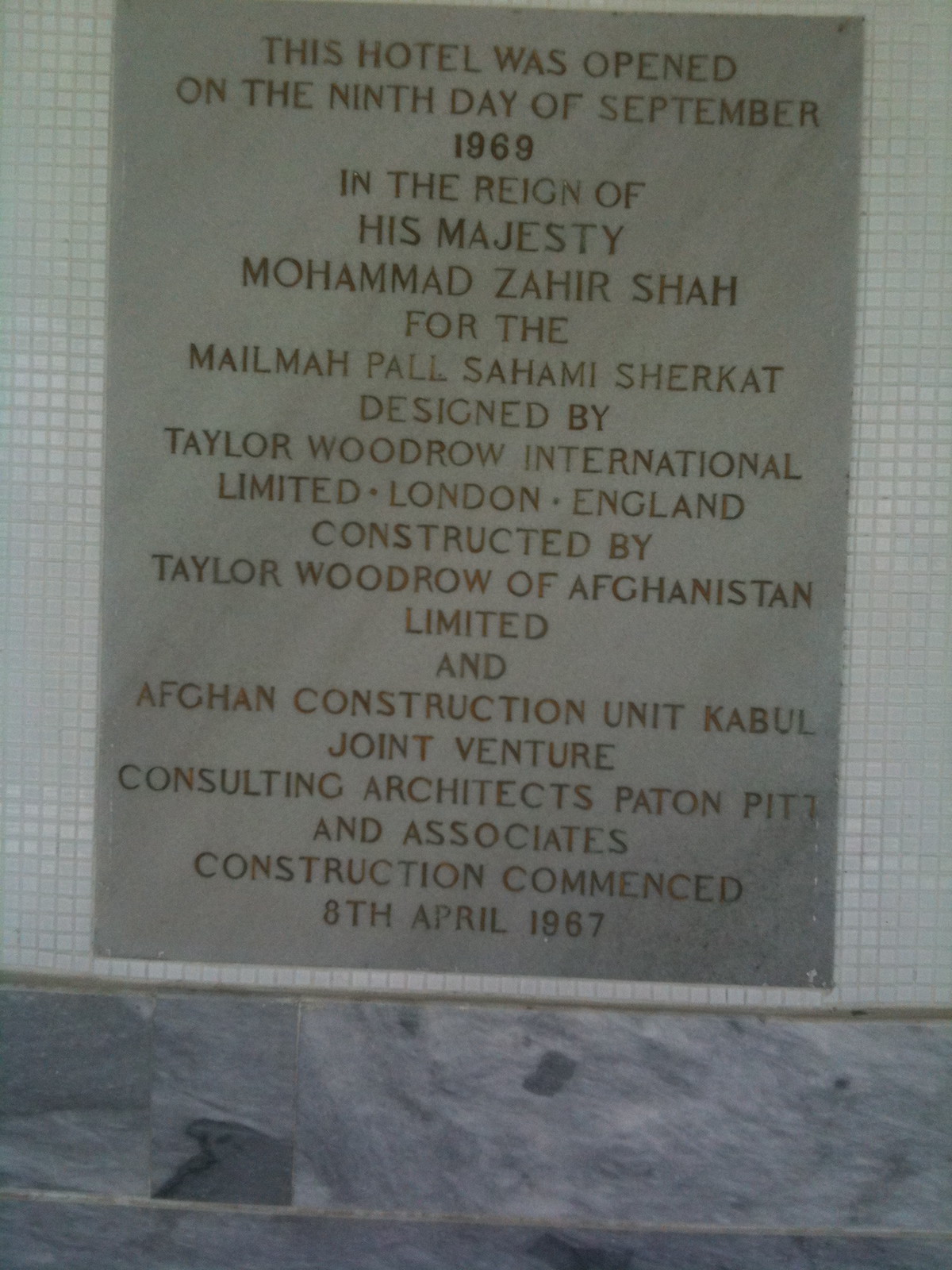The image showcases a commemorative plaque affixed to a wall, prominently positioned above a marble slab trim. The plaque, composed of a small square white tile, features dark brown etched text. It reads: "This hotel was opened on the 9th day of September 1969 during the reign of His Majesty Mohammed Zahir Shah for the Malma Paul Sahani Shukat. It was designed by Taylor Woodrow International Limited, London, England, and constructed by Taylor Woodrow of Afghanistan Limited and Afghan Construction Unit, Kabul Joint Venture Consulting Architects Patan Pitwan and Associates. Construction commenced on the 8th of April 1967." The backdrop appears to be dark gray, possibly resembling marble, adding to the plaque's elegant presentation.